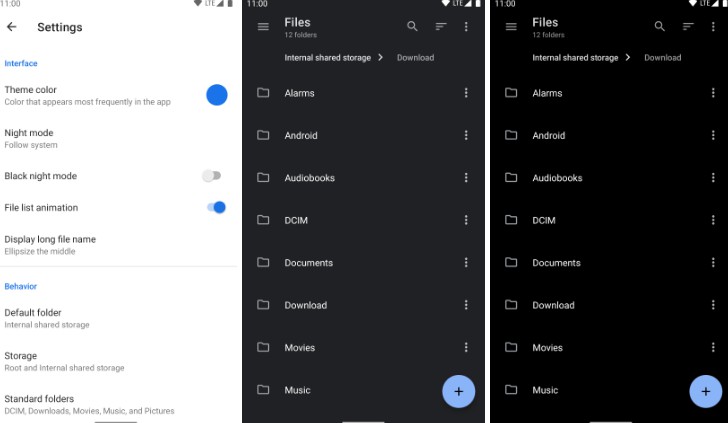The image is a collage composed of three distinct sections. 

On the left side, the topmost part displays a time of "11:00" followed by the word "Settings" beneath it. Below "Settings," there is a blue text labeled "Interface" and a black text that says "Theme Color," describing "Color that appears most frequently in the app."

Next to this brief description, there is a blue circle. Below this, there are options for "Night mode: Follow System," followed by "Black Night Mode," with an on/off switch set to the right. Further down is an option for "File List Animation," also accompanied by an on/off switch which is turned on. Below that is an option titled "Display Long File Name," and further below, there's a section labeled "Behavior" in blue text. This section includes three grey options: "Default Folder," "Storage," and "Standard Folders," each accompanied by a small line of explanatory text.

The middle section features a black background with white text at the top that reads "Files." Directly beneath this, it says "Internal Shared Storage," followed by a list of folders ordered from top to bottom. These folders include "Alarms," "Android," "Audiobooks," "DCIM," "Documents," "Download," "Movies," and "Music."

On the right side, the section mirrors the middle part, showing another file interface with identical folders listed in the same order: "Alarms," "Android," "Audiobooks," "DCIM," "Documents," "Download," "Movies," and "Music."

The overall layout of the image appears to showcase a settings interface for an application, emphasizing customization options and a detailed file management system.